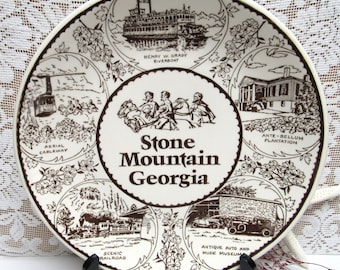The photo showcases an oval-shaped commemorative plate held by a small black stand, set against a lacy, floral-patterned background, likely a doily or tablecloth. The plate, rendered in black and white, prominently features the text "Stone Mountain, Georgia" in three separate lines at its center, surrounded by a scalloped black circle. Below the text, there is a drawing in pen and ink of what appears to be three or four people and two horses, although the image is somewhat blurry. Additionally, five circular illustrations, representing tourist attractions in Stone Mountain, Georgia, decorate the outer ring. These include an aerial cableway with a cable car, a scenic railroad with a train, an antique auto museum depicting classic cars in front of a building, an antebellum plantation house surrounded by plants, and at the very top, the Henry W. Grady riverboat. The illustrations are detailed in a simple, monochromatic style, contributing to the plate's intricate and nostalgic design.